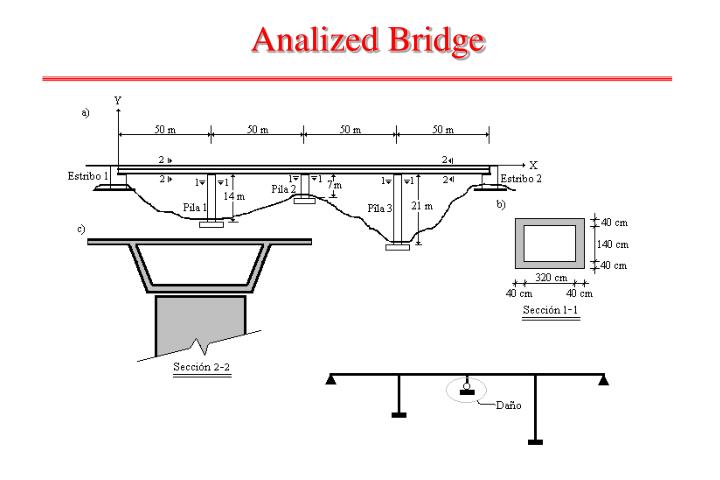The image is a detailed technical diagram of a bridge design, likely intended for engineers. Dominated by a red title reading "Analyzed Bridge" (spelled A-N-A-L-I-Z-E-D) across the top, the image features an underline beneath the title. The primary portion of the diagram includes a series of labeled schematics and graphs centered around a bridge structure. Notably, one axis of a graph includes the Spanish word "Estadible," indicating a potential multilingual aspect.

The diagram is divided into several sections:
- **Section A**: Labeled "Estribo 1," it includes various measurements, presumably of a structural component.
- **Section B**: A rectangle with measured heights of 40 cm, 140 cm, and widths ranging from 40 cm to 320 cm, labeled "Section 1-1."
- **Section C**: Depicts a trapezoid-shaped image labeled "Section 2-2." 
- **Section D**: Features a horizontal line intersected by two vertical lines, focusing on an area labeled "Daño" (with a tilde over the 'n'), which translates to "damage" in English.

Additional graphical elements include multiple plots and data graphs. One graph, metricized in meters, spans from 50m across four quadrants, with two notable peaks in the first and third quadrants. Other measurements range between 40 cm, 140 cm, and 240 cm, depicting various structural dimensions.

Overall, the image illustrates a comprehensive schematic of the bridge’s measurements and sections, designed to convey intricate engineering details.